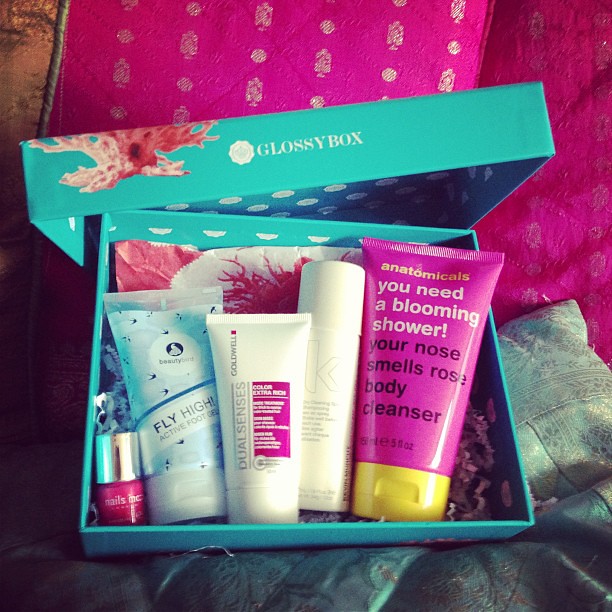The photograph showcases an aqua blue box with a polka dot design on the inside, possibly designed with a floral or coral-like print. The lid of the box, which is leaning against the back, features the logo "GlossyBox" prominently. The box is nestled among pink velvet and blue pillow backgrounds, suggesting it might be placed on a sofa or bed. Inside the box, cradled in crinkly paper confetti, are five beauty and self-care products. On the far left is a hot pink nail polish bottle. Next to it is a tube labeled "Fly High Active Foot Gel." The middle item appears to be a tube from the "DualSenses Color Extra-Rich" line, possibly a conditioner or shampoo. There's another white bottle with a barely visible 'K' on it. Finally, on the right side is a pink bottle with a yellow cap that reads, "Anatomicals: You Need a Blooming Shower, Your Nose Smells Rose," a body cleanser. The meticulous arrangement of these varied beauty products contributes to an overall sense of luxury and self-care.